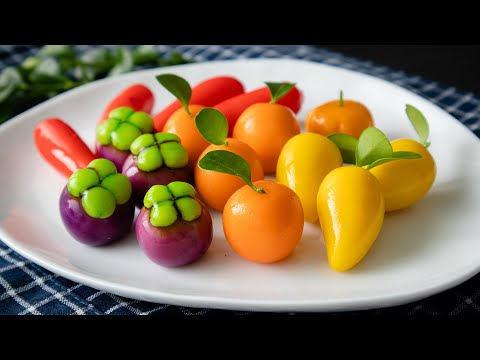This detailed color photograph, in landscape orientation, captures a meticulously arranged selection of glossy ceramic fruit shapes displayed on a white round plate. The plate rests on a blue and white checkered cloth that covers the entire table. The vibrant fruit creations—including purple plums, each adorned with a green four-leaf top (four in total), five round oranges with individual green leaves, and a yellow pear-like shape with a green leaf—along with four orange, short tube-like objects that might resemble carrots, are positioned harmoniously on the plate. Each fruit shape is crafted to a high gloss finish, suggesting a hand-painted design by an artist, contributing to the overall aesthetic. The photograph's representational, realistic style is further emphasized by a horizontal black stripe at the top and bottom of the image.